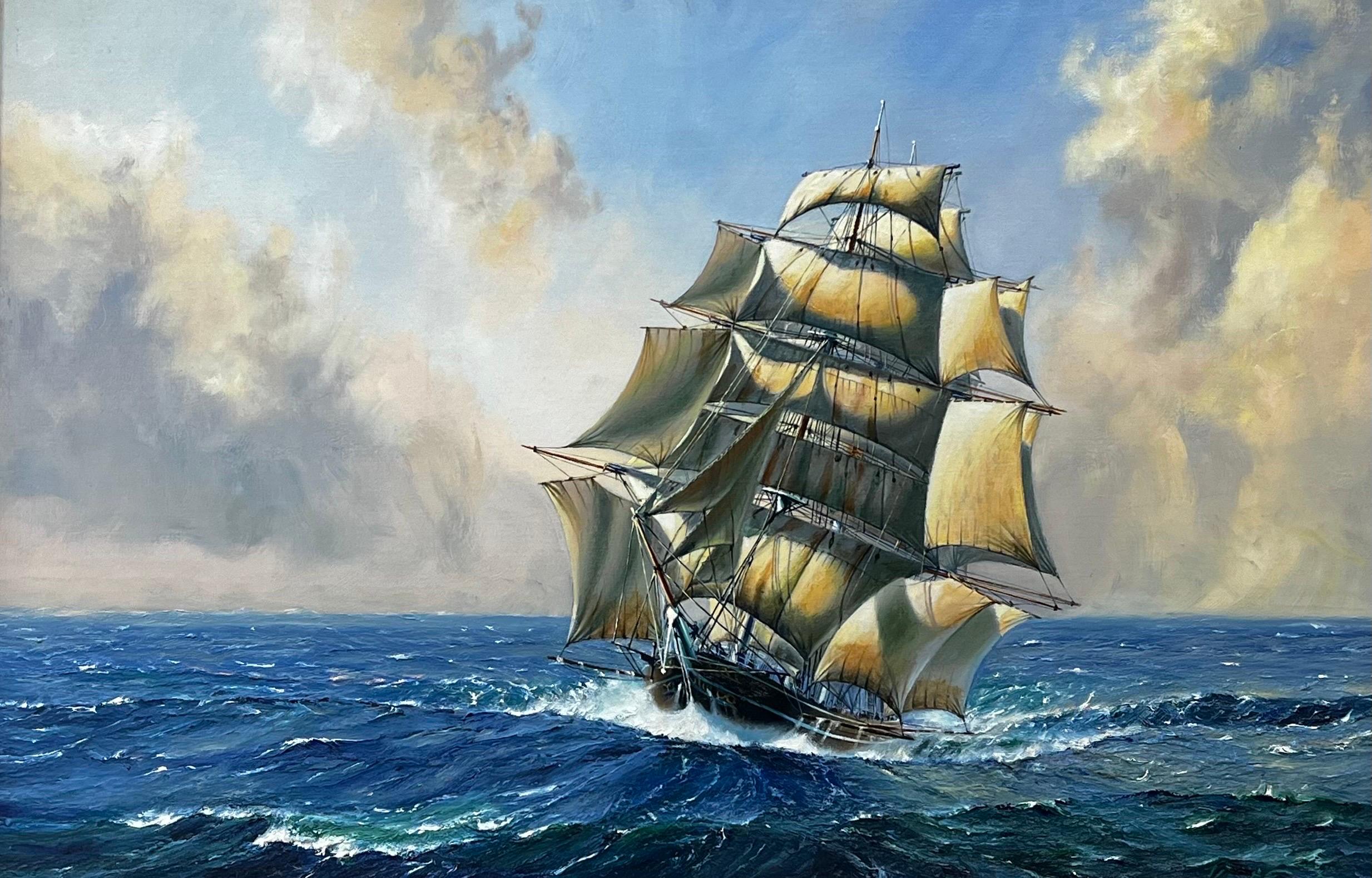The painting depicts a large, brown wooden clipper ship sailing on a tumultuous blue ocean with aqua-colored waves and white breakers. The ship, slightly right of center and facing left, is adorned with myriad sails; the bottom tier has six horizontal sails, the next tier features eight, further up there are four, and the very top carries two wide, narrow sails. The deck is bustling with people, noticeable by the tiny specks scattered across it. The sky above is a mix of light blue patches and looming cumulus clouds tinged with gray and purple hues, suggesting a stormy ambiance. The wind is strongly blowing, evident from the full, unfurled sails. The detailed painting, with a realistic touch, captures the dynamic motion of the ship as it tips slightly, cutting a wake through the rough sea.